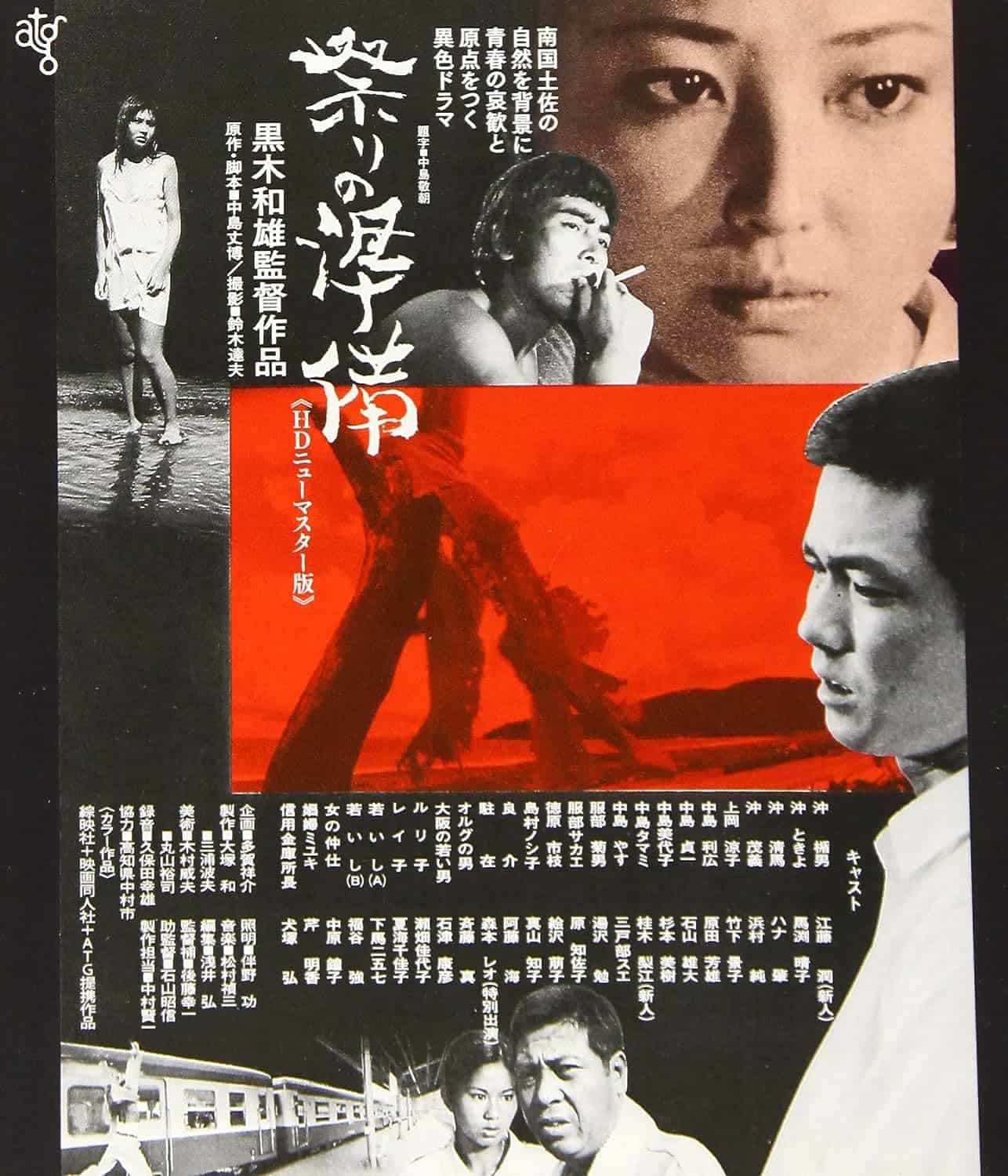The poster, likely for an Asian film, seems to be in Japanese, displaying vivid and detailed imagery. In stark black and white, one protagonist—a man—sits pensively, smoking a cigarette. Behind him, a young, wide-eyed woman stands in a contemplative pose. Below, another scene showcases this woman, barefoot in a white outfit, playing in a puddle of water, with a bewildered young man nearby. Dominating the poster is an intense central image of characters, possibly these protagonists, engaging in a battle against a fiery red dragon-like monster. The background suggests a coastal scene, merging both fantasy and everyday elements. At the bottom, a couple appears poised to board a train, adding a layer of intrigue and suggesting a narrative steeped in mystique, action, and drama.